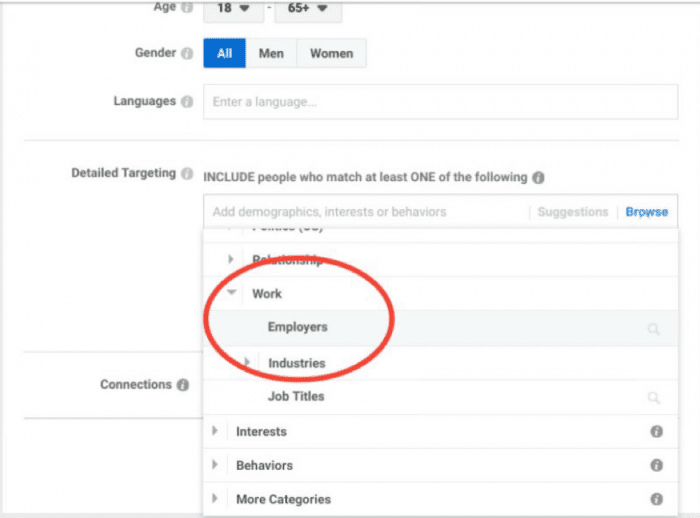This image is a screen capture from a computer displaying a segment of an online form or application for targeted advertising. The top section is labeled "Age," featuring a dropdown menu with options "18" (with a down arrow) and "65+" (with a down arrow). Below this, the "Gender" section shows a blue rectangle indicating "All," followed by a gray rectangle for "Men" and another gray rectangle for "Women."

The next section is "Languages," with a fine print prompt reading "Enter a language." Beneath "Languages," the "Detailed Targeting" section begins with the capitalized word "INCLUDE," followed by the instruction, "People who match at least one of the following." Below this, there is an option to "Add demographics, interests, or behaviors," accompanied by a "Suggestions" area and a "Browse" button.

Prominently marked in the "Detailed Targeting" section is "Work," highlighted by a digitally added red or egg-shaped circle. Subcategories under "Work" include "Employers" and "Industries."

Further down, the form includes sections for "Connections," "Job Titles," "Interests," "Behaviors," and "More Categories." These areas offer additional criteria for fine-tuning the ad targeting further.